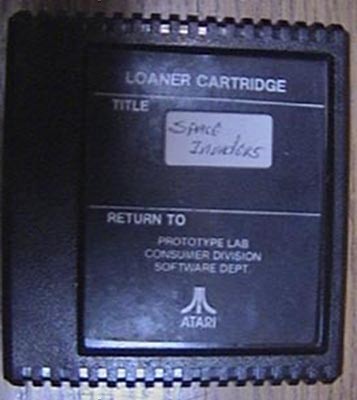This color photograph captures a detailed image of a vintage cartridge, possibly from a gaming console, set against a contrasting dual-colored background. The main subject, the cartridge, prominently occupies the central frame and is distinctly characterized by a dark grey body with serrated edges at the top and bottom. The background features a lighter grey surrounding on the top, right, and bottom sides, enhancing the contrast and drawing the viewer's attention to the cartridge itself.

Notably, the cartridge displays reflective holes, suggesting a metallic or glossy material. Its rectangular design casts a shadow toward the upper left corner, adding a touch of depth to the image. The cartridge is adorned with white text that reads "Loaner Cartridge" at the top, followed by a thin horizontal line. Below this, there is a title encased within a white rectangle, featuring black writing that remains unreadable. Another horizontal line follows, leading to more white text stating "Return to Prototype Lab, Consumer Division, Software Department."

At the center of the lower half of the cartridge, there's a small logo resembling a mountain shape with a curved middle, accompanied by the word "Atari" underneath. A subtle light reflection is also visible towards the bottom left corner of the cartridge, further accentuating its glossy finish. The meticulous details and reflective elements bring this vintage technology to life, making it a captivating and nostalgic subject.